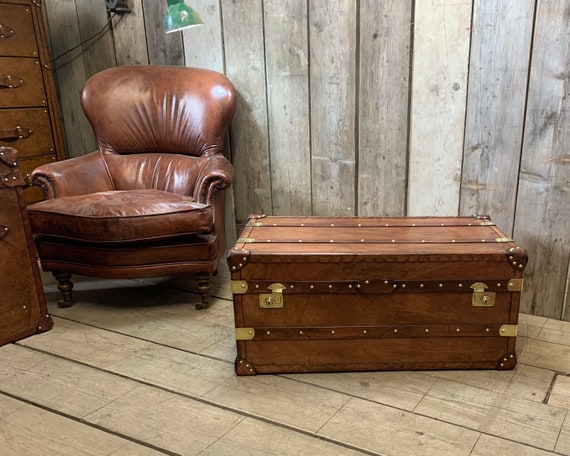The photograph showcases a cozy room inside a wood cabin adorned with wooden panel walls and a wooden floor. Central to the scene is a vintage, brown leather chair paired with a wooden and leather chest of drawers, both exuding a rich brown hue. Accompanying these pieces are two brown leather trunks, highlighted with gold or brass tacks, adding a touch of elegance. These vintage furnishings are complemented by a green hanging lamp that casts a warm light over the space, waiting for its inhabitant. The overall ambiance of the room suggests it could be either a bedroom or a living room, offering a rustic charm with its smoky gray and brown tones and vertical wooden wall panels.